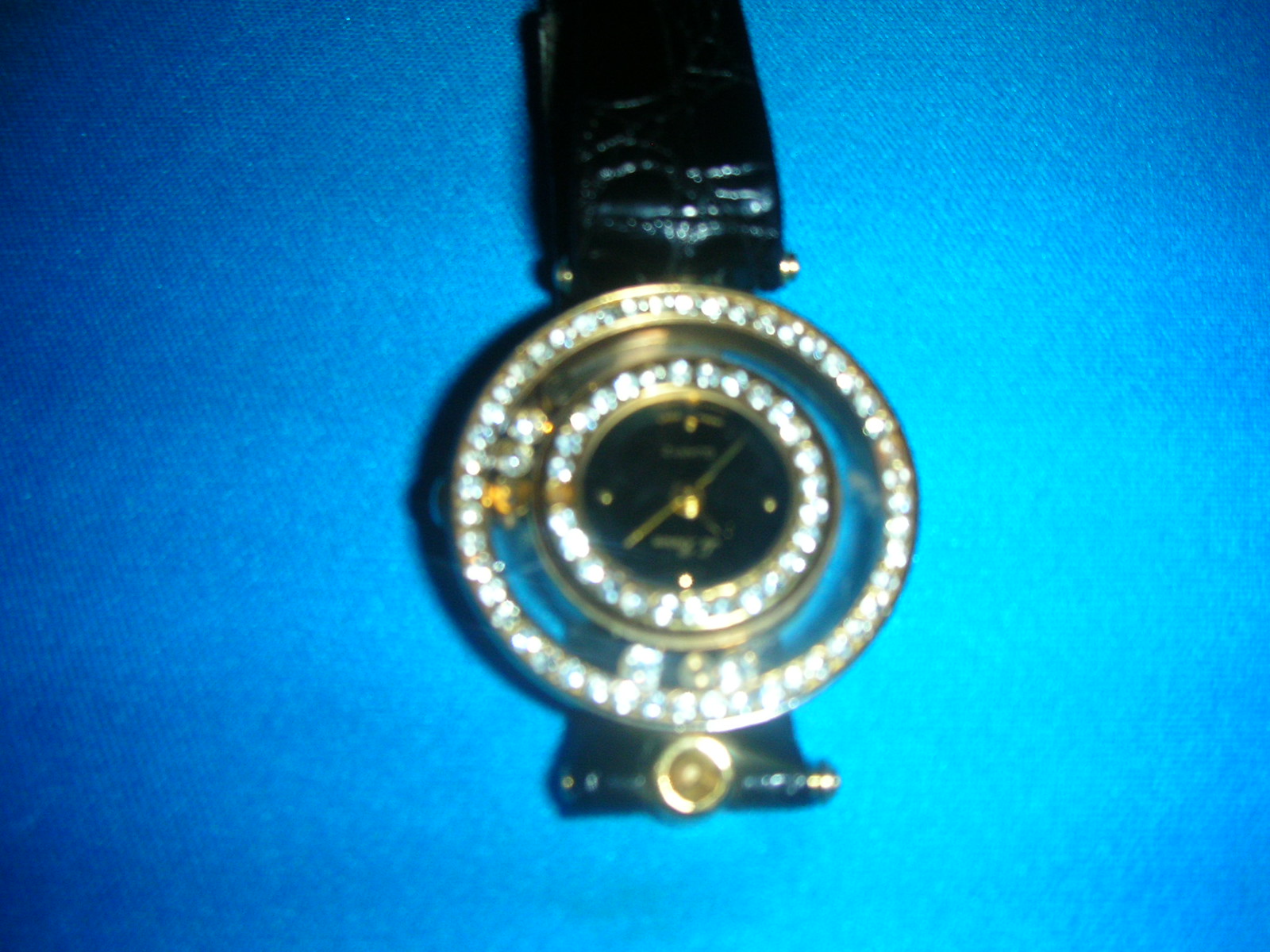This image depicts an exquisite, avant-garde wristwatch characterized by its distinctive and abstract design. The watch features two circular, golden rings encrusted with small, sparkling diamonds, which are elegantly encased in what appears to be glass. At the center of these interlocking rings lies a smaller, black watch face adorned with four golden markers, providing a minimalist yet striking appearance. The watch face is equipped with two golden hands indicating hours and minutes. The luxurious aesthetic is further enhanced by a finely crafted leather band, adding a touch of sophistication. The entire assembly is artistically presented against a rich, blue felt backdrop, accentuating the watch’s opulence and intricate detailing.